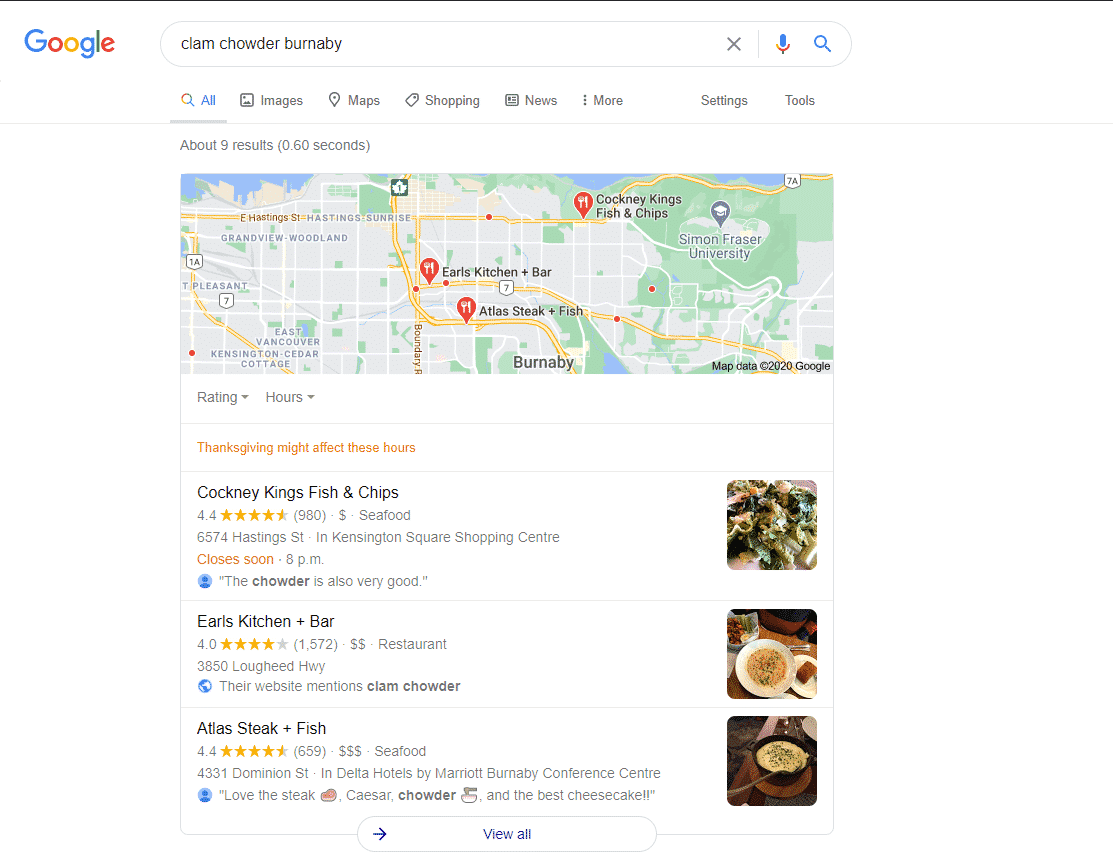This image is a screenshot of a Google search results page for "clam chowder Burnaby." The familiar Google logo is situated in the top left corner. Directly below, the search bar displays the query and is flanked by an 'X' to clear the search, a microphone icon for voice search, and a blue search button. Beneath the search bar, there is a navigation bar with tabs labeled "All," "Images," "Maps," "Shopping," "News," and "More." To the far right, options for "Settings" and "Tools" are visible.

Directly below this, it mentions "About 9 results" which were found in 0.60 seconds, followed by a map visually marking several locations in Burnaby with pins. The identified locations include Cockney Kings Fish & Chips, Earls Kitchen + Bar, Atlas Steak + Fish, and an additional pin for Simon Fraser University, indicating the general area of Burnaby.

Further down, there are drop-down boxes for user ratings and business hours, noted with an advisory in orange stating, "Thanksgiving might affect these hours." Listings for the mentioned places appear below, each accompanied by a thumbnail image to the right, providing a visual reference for the entries.